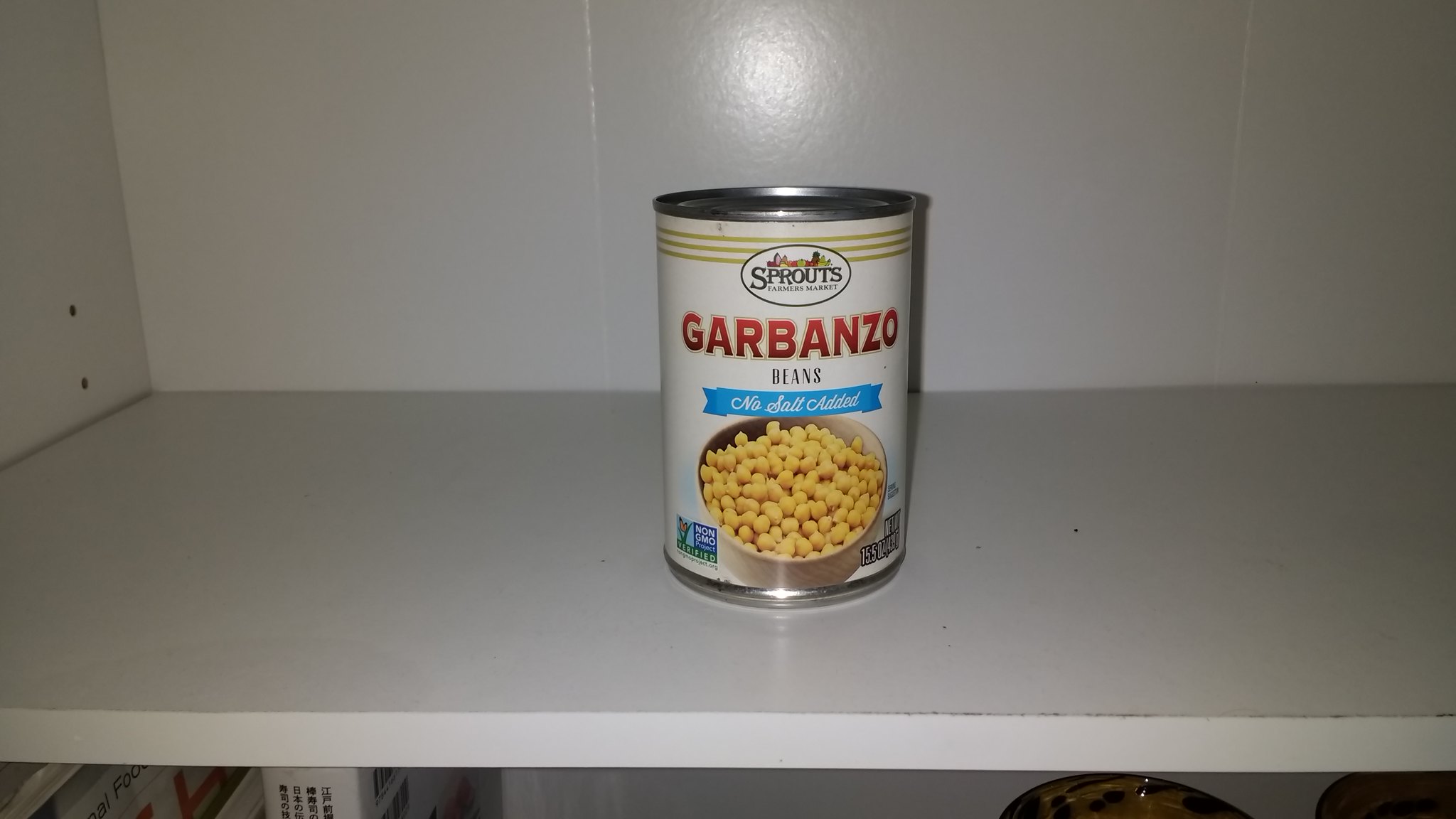The image depicts a single shelf within a stark white cabinet, which, due to the lighting, appears to have a delicate pale lilac hue. An overhead light or camera flash causes a reflective gleam on the back wall. Centered on the shelf is a can prominently displaying "garbanzo" in bold red letters, with "beans" noted beneath in smaller text and the phrase "No salt added." The label features a horizontally-aligned oval with the company name, partially readable as "something sprouts." The label's background is white, accented by three golden lines encircling the top. On the right side of the can is a weight indication, possibly reading "15 oz," and to the left is a small blue square labeled "non-GMO." In front of the can is a bowl filled with tan garbanzo beans. The top of the next lower shelf is faintly visible but its contents are indiscernible.